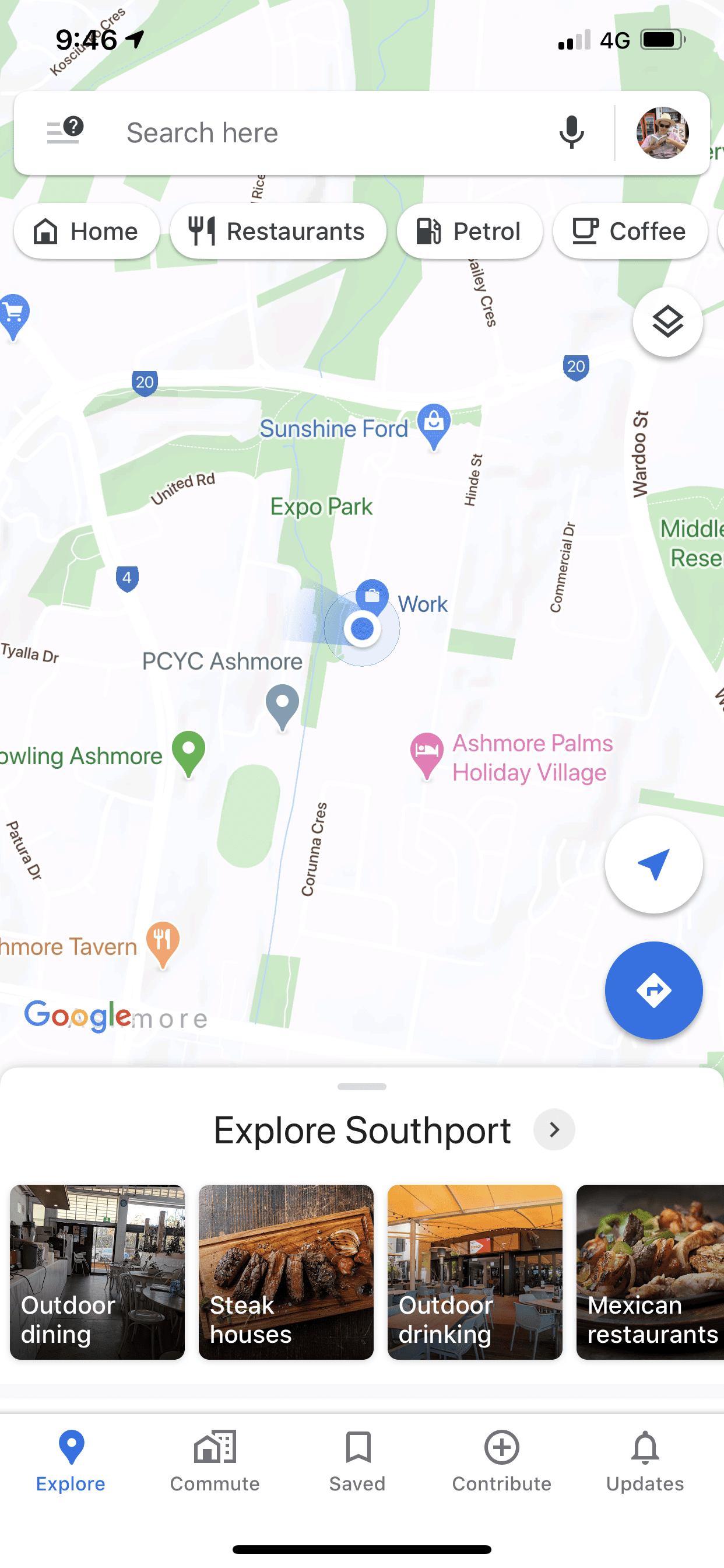This image is a screenshot of Google Maps, showcasing the current location of an individual. Centered on the map is a blue location dot with a semi-northwest pointing gradient radiating from it, indicating the direction the device is facing. At the top of the screen, there is a search bar alongside the person's profile icon, presumably a picture of them.

Just below the search bar, a row of capsule-shaped buttons marked in white offers quick access to categories such as Home, Restaurants, Petrol, and Coffee. The use of the term "petrol" suggests that the person is not located in the United States.

Several landmarks are displayed on the map, including Sunshine Ford, Ashmore Palms Holiday Village, PCYC Ashmore, Ashmore Bowling, and Ashmore Tavern. At the bottom of the screen is a pull-up panel, identifiable by a small gray horizontal handle at the top.

The panel comprises sections titled "Explore Southport," denoted by a right-facing arrow inside a gray circle. Underneath are various categories with representative images: "Outdoor Dining" shows an indoor restaurant scene, "Steak Houses" features slices of medium-rare steak on a wooden carving board, "Outdoor Drinking" depicts the interior of a yellow tent with seating arrangements, and "Mexican Restaurants" displays a plate of fajitas.

Further down is a menu with options labeled Explore (highlighted in blue, indicating the current view), Commute, Saved, Contribute, and Updates.